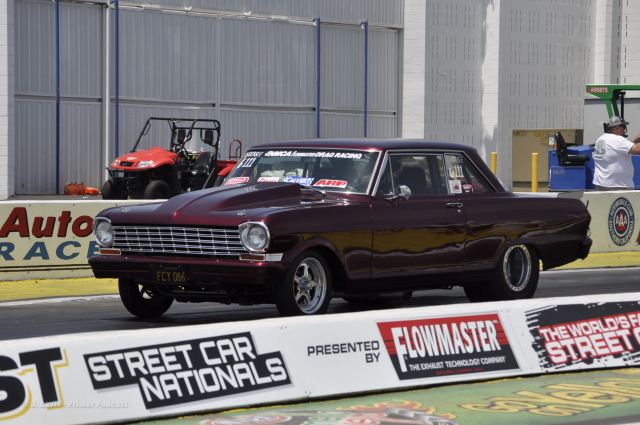This image captures a vintage muscle car, likely from the 1960s or 70s, on a racetrack. The car is a vivid purple with a burgundy hue and features a large hood and distinct small front wheels paired with large back wheels, indicating modifications for street racing. The windshield carries several decals, including "Drag Racing" and "ARP," among other advertisements. In the foreground, banners prominently display "Streetcar Nationals, presented by Flowmaster" amidst additional text, "the world's best speed race." The backdrop includes a red ATV and a man in a white t-shirt near what appears to be a warehouse. The scene suggests the car is primed for a high-speed run, exuding the aura of power and noise typical of classic muscle cars.